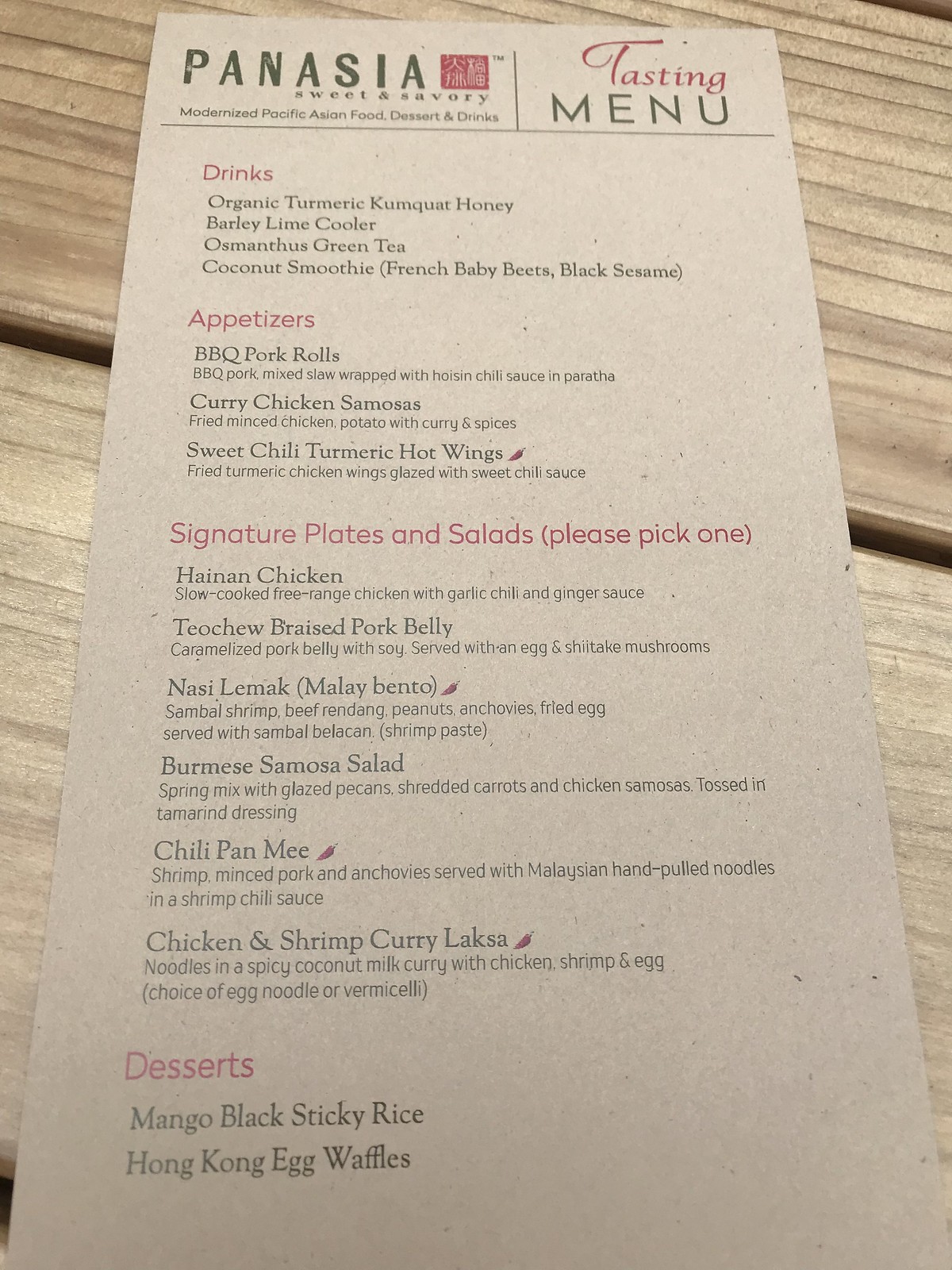The image is a detailed tasting menu set against a tan-colored wooden table with horizontal stripes. The menu prominently occupies the majority of the image. The top left corner of the menu features the restaurant name, "PANASIA," in capital letters, followed by the tagline "sweet and savory" in lowercase text. Below this, it states, "modernized Pacific Asian food, dessert, and drinks." 

In the top right corner, "tasting menu" is prominently displayed with the word "tasting" in red letters. Below it, the "drinks" section is labeled in red text, featuring the following options in black letters:
- Organic Turmeric Kumquat Honey
- Barley Lime Cooler
- Osmanthus Green Tea
- Coconut Smoothie (French baby beets, black sesame)

The next section, titled "appetizers" in red text, lists:
1. BBQ Pork Rolls - BBQ pork mixed with slaw, wrapped with hoisin chili sauce in paratha.
2. Curry Chicken Samosas - Fried minced chicken and potato with curry and spices.
3. Sweet Chili Turmeric Hot Wings - Fried turmeric chicken wings glazed with sweet chili sauce.

Under "signature plates and salads" (please pick one), with the section title in red, the selections include:
- Hainan Chicken: Slow-cooked free-range chicken with garlic chili and ginger sauce.
- Teochew Braised Pork Belly: Caramelized pork belly with soy, served with an egg and shiitake mushrooms.
- Nasi Lemak (Malay bento): Sambal shrimp, beef rendang, peanuts, anchovies, fried eggs, served with sambal belacan (shrimp paste).
- Burmese Samosa Salad: Spring mix with glazed pecans, shredded carrots, and chicken samosas tossed in tamarind dressing.
- Chili Pan Mee: Shrimp, minced pork, and anchovies served with Malaysian hand-pulled noodles in shrimp chili sauce.
- Chicken and Shrimp Curry Laksa: Noodles in a spicy coconut milk curry with chicken, shrimp, and an egg (choice of egg noodle or vermicelli).

Lastly, the "desserts" section in red text offers:
- Mango Black Sticky Rice
- Hong Kong Egg Waffles